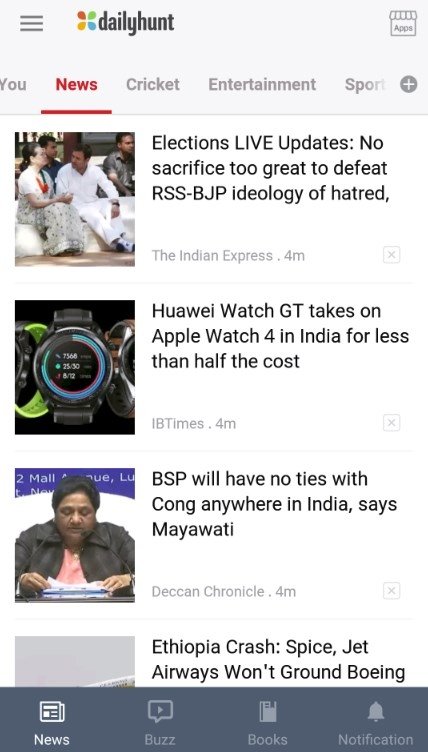The image depicts a user interface of the Daily Hunt app, a news aggregation platform popular in India. The app's top navigation bar features a hamburger menu on the left, and the Daily Hunt logo—a stylized flower with four teardrop-shaped petals in green, blue, yellow, and red. On the right, there's an icon for the app store.

Below the navigation bar, users can select different categories: "You," "News," "Cricket," "Entertainment," and "Sports." Here, the "News" category is highlighted in red, indicating it is currently active. Four headlines with accompanying images are prominently displayed:

1. The first headline, from the Indian Express, reports on elections with the title, "Live Update: No sacrifice too great to defeat RSS-BJP ideology of hatred," dated four minutes ago. The adjacent image shows a man in a white suit seated next to a woman in a dress.
   
2. The second story discusses technology, spotlighting the Huawei Watch GT's competition with the Apple Watch 4 in India, emphasizing its lower cost. 

3. The third headline from the Deccan Chronicle reports on politics, with the title, "BSP will have no ties with Kong anywhere in India, says Maya Wadi," also reported four minutes ago. The accompanying image shows a person reading while facing the camera.

4. The fourth headline, partially obscured, mentions a crash in Ethiopia involving SpiceJet Airways and Boeing aircraft.

At the bottom of the app's interface are navigation icons for "News," "Buzz," "Books," and "Notification." The "News" section is currently selected, represented by a newspaper icon. The other icons are grayed out: "Buzz" has a speech bubble, "Books" displays an open book, and "Notification" features a bell.